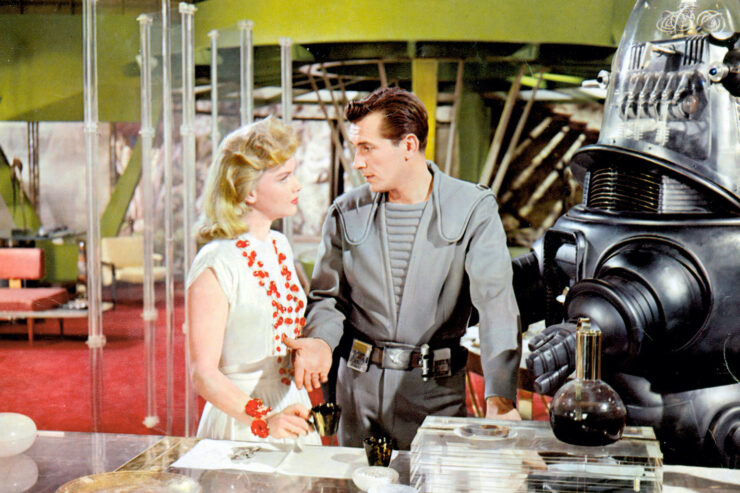The image appears to be a colorized or color TV still from a sci-fi show, potentially "Buck Rogers" or "Lost in Space." In the center stands a man and a woman. The man, possibly Buck Rogers, is dressed in a futuristic gray space explorer suit featuring droopy lapels and a ribbed neck extending to his navel. His outfit is complemented by a utility belt adorned with various compartments, and he has dark brown slicked-back hair. He appears to be in conversation with a woman standing closely beside him. 

The woman sports a 60s-style white sleeveless dress paired with a multi-stranded red beaded necklace and a matching bracelet. She has medium-length blonde hair and noticeable makeup, including red lipstick. 

To the right of the duo is a distinctive black robot resembling an upright beetle, with a clear glass head revealing internal gears and mechanisms. Behind them is a circular roof structure featuring concentric circles and radial beams, rendered in a yellowish-green hue. The background is complemented by a red carpet and mid-century modern furniture, including both armchairs and armless chairs. On a nearby table, there's a mid-century coffee carafe and small cups, adding to the retro-futuristic ambiance of the scene.